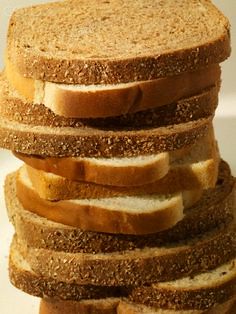This indoor color photograph features a close-up, vertical stack of approximately 11 to 12 slices of bread, alternating between white and wheat varieties. The stack is slightly twisted to the left and right, creating a disordered appearance. The top slice is darker and rougher, likely wheat or rye, revealing visible grains and holes. The bread appears lightly toasted. The background is an indistinct, out-of-focus off-white or light gray, with slightly darker tones on the right side, indicating a light source from the left. The edges of the bread, particularly on the left, extend slightly out of the frame, emphasizing the vertical orientation of the image.